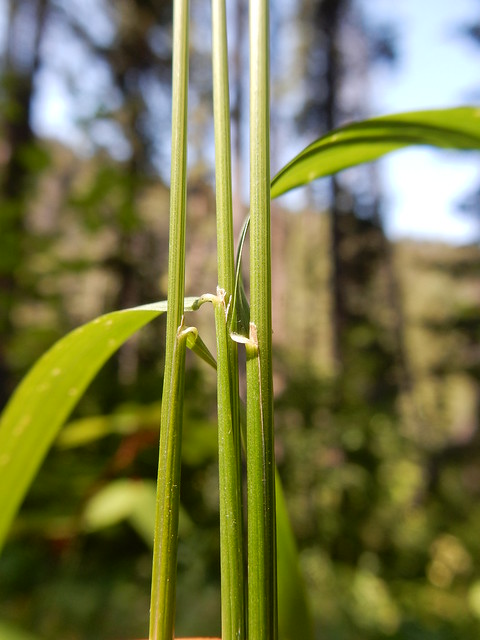The image features a detailed close-up of a vibrant green plant, showcasing three tall, straight stalks that dominate the frame by growing vertically, filling the entire image. There are two leaves sprouting from these stalks, adorned with lighter or yellow speckles. The leaves hang off the stalks, appearing intermittently. The backdrop, while blurry, hints at a lush garden or woodland scene, bathed in the bright, saturated colors of a sunny day. A faint blue sky is visible behind a possible garden fence, adding to the serene outdoor setting. The photographer has emphasized the long, straight stalks and the intricate details of the leaves, presenting a focused and immersive view into a lively corner of nature.